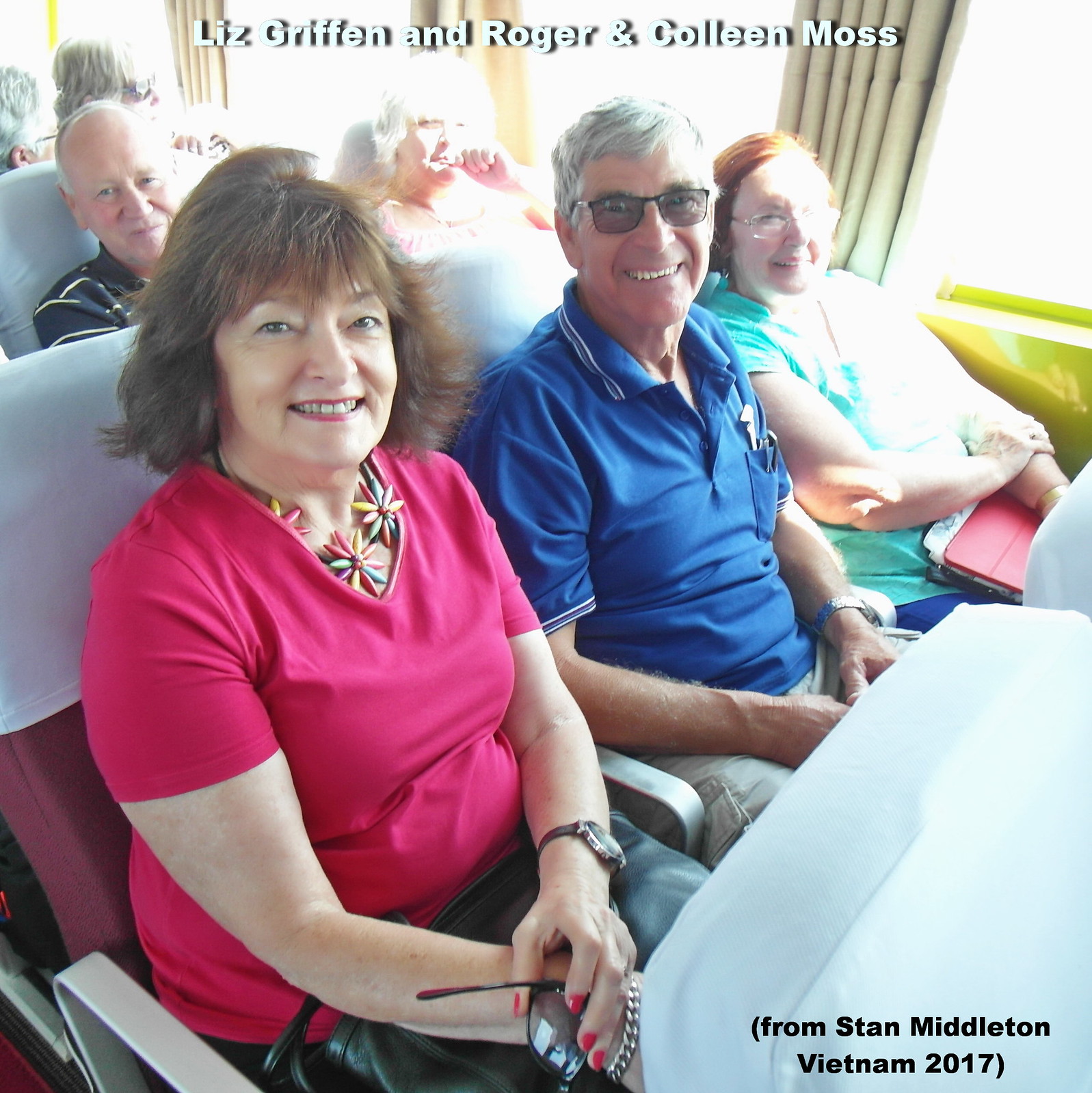This is a detailed photographic image set inside what appears to be a train, featuring a group of elderly white individuals. At the forefront, seated in a row of train seats, are three people: a white woman wearing a pink top and a floral necklace, a white man in a blue shirt and khaki pants, and a white woman in a turquoise short-sleeved shirt clutching what seems to be a laptop or a tablet. The man is also wearing sunglasses. Behind them, another row holds an elderly white couple; the man has balding black and white hair and wears a black shirt with white stripes, while the woman, also elderly and white, is dressed casually. The background includes the tops of heads from other passengers. At the top center of the image, the text "Liz Griffin GRI FF EN and Roger and Colleen Moss" is prominently displayed in white, outlined in black. The bottom right corner of the image contains the text "from Stan Middleton Vietnam 2017," providing context to the setting and date of the photograph.